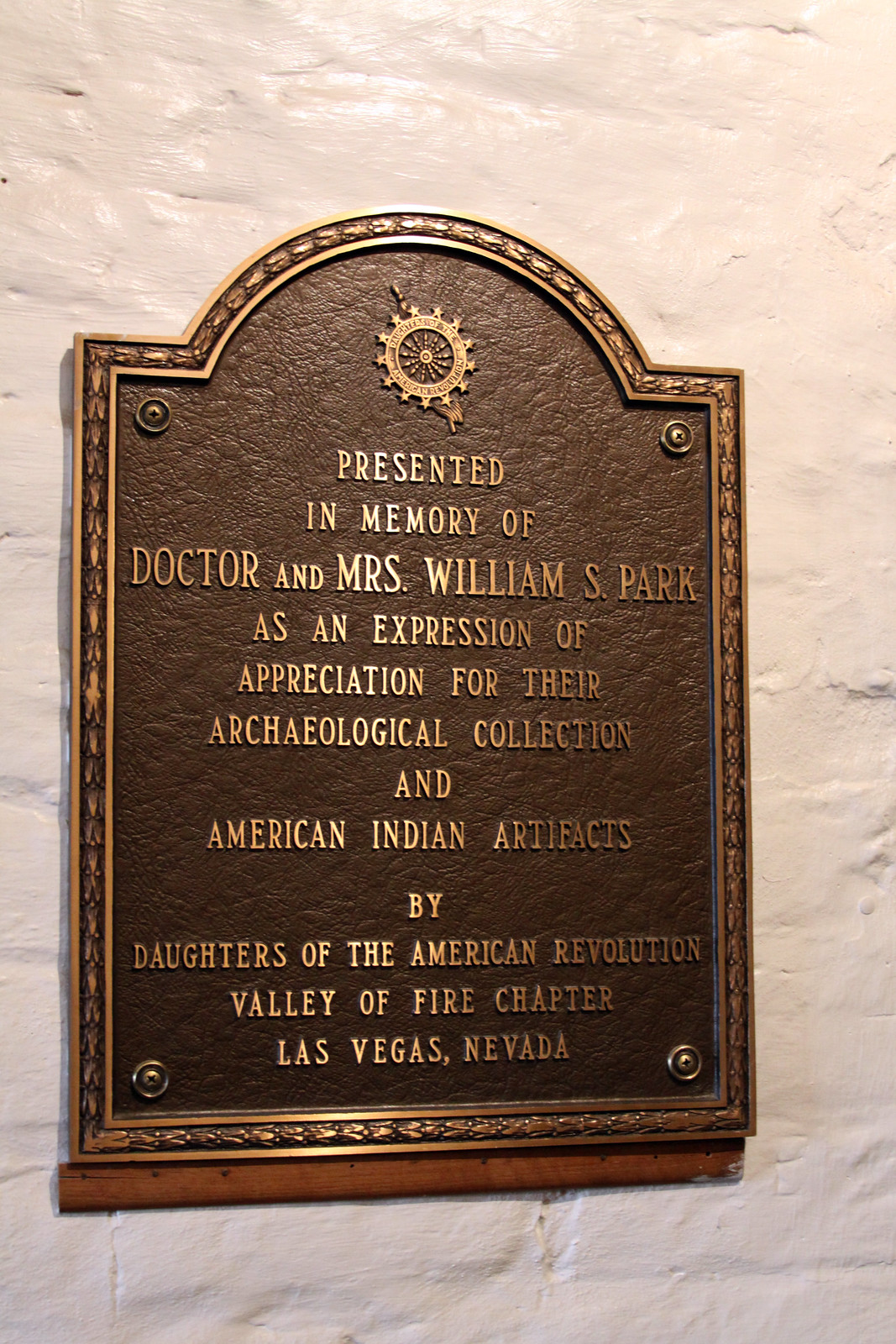The image displays a commemorative plaque set against a white plastered wall with a residue of brick texture faintly visible beneath. The plaque, which has a textured brown surface resembling brown leather, is encased in a golden frame with golden letters. Positioned in the top center of the plaque is an insignia or emblem associated with the Daughters of the American Revolution. Below this logo, the text reads: "Presented in memory of Dr. and Mrs. William S. Park as an expression of appreciation for their archaeological collection and American Indian artifacts by the Daughters of the American Revolution, Valley of Fire Chapter, Las Vegas, Nevada." The plaque hangs centrally on the wall, slightly to the left within a vertical photograph. Below the plaque, there is a wooden support also attached to the wall. The overall setting has an old, historic feel, suggesting it might be related to an archaeological site.